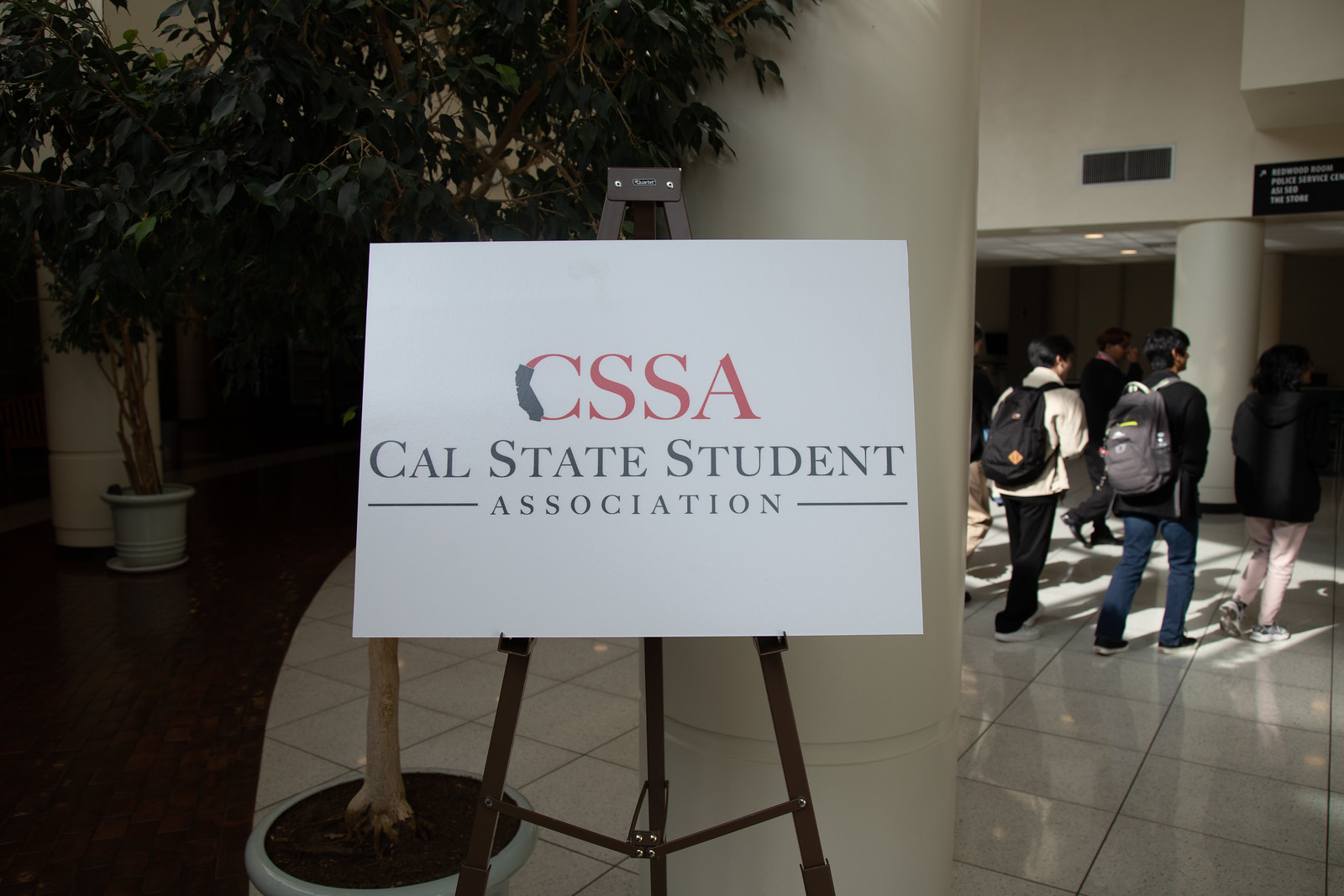This photorealistic image, taken indoors, captures a scene likely at a convention center or similar venue. Central to the image is a white rectangular sign on a brown easel-style holder. Prominently displayed in bold red, capital letters are “CSSA,” with "Cal State Student Association" detailed below in a darker blue or gray font. To the left of the sign, a green-leaved tree in a gray pot is partially visible, with another similar tree in the distant background. A white column stands immediately behind the sign. The flooring transitions from dark brown on the left side of the image to a clean, shiny white or light gray tile with dark grout on the right. Several students, carrying backpacks and dressed in casual attire, walk towards the right side of the frame, adding a sense of movement through the well-lit, white-walled space.